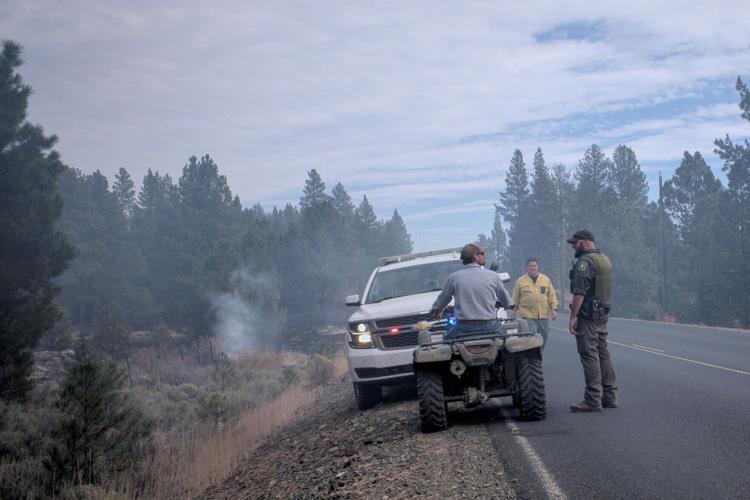The photograph captures a scene on a forested road featuring a park ranger interaction. A Caucasian man on an ATV is positioned with his right wheel on the road and his left wheel on the dirt shoulder. The man wears a gray shirt, brown baseball cap, and sunglasses. His back is to the camera as he looks towards a park ranger standing to his right. The ranger is dressed in a greenish uniform with a baseball cap and various utility items on his belt, potentially including a walkie-talkie. Approaching them from the background is another man in a yellow long-sleeved shirt and blue jeans. Directly in front of the ATV, facing the man on it, is a white Chevrolet pickup truck equipped with flashing siren lights. The truck's positioning suggests an ongoing interaction or checkpoint. Surrounding the scene are tall pine trees, and the sky above is mostly cloudy with hints of blue peeking through. The atmosphere appears slightly smoky or hazy, potentially indicating the presence of a distant fire in the wooded area.